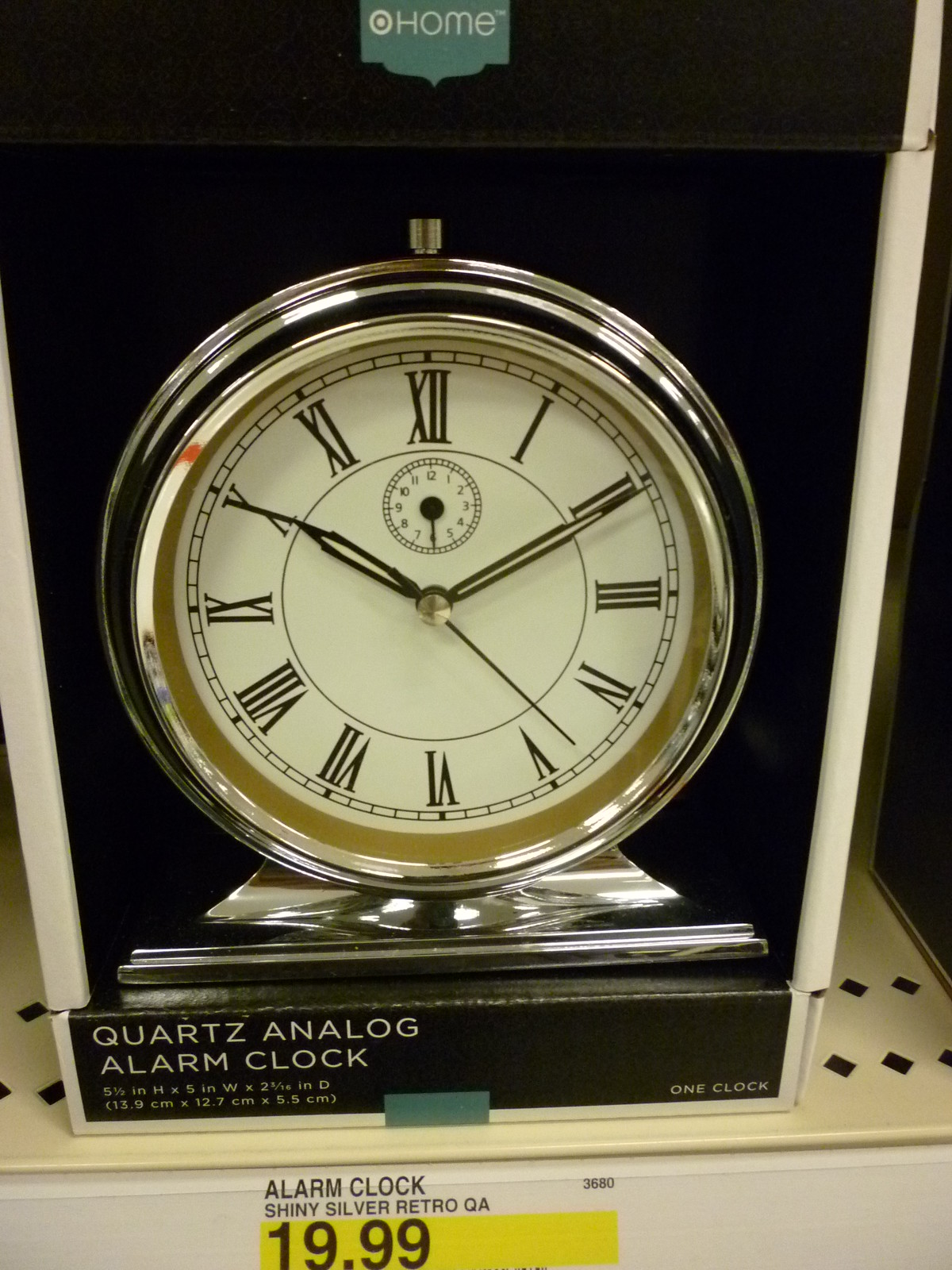In this image, we are inside a store, focusing on a boxed Quartz Analog Alarm Clock. The clock has a shiny silver finish with a retro design, featuring Roman numerals on its face. The packaging is sleek, predominantly black and white, and is designed to allow a clear view of the clock within. This clock is freestanding, meant to sit on a surface rather than being mounted on a wall. The dimensions of the clock are specified as 5 1/2 inches in height, 5 inches in width, and 2 1/16 inches in depth. A visible price tag indicates it is selling for $19.99.